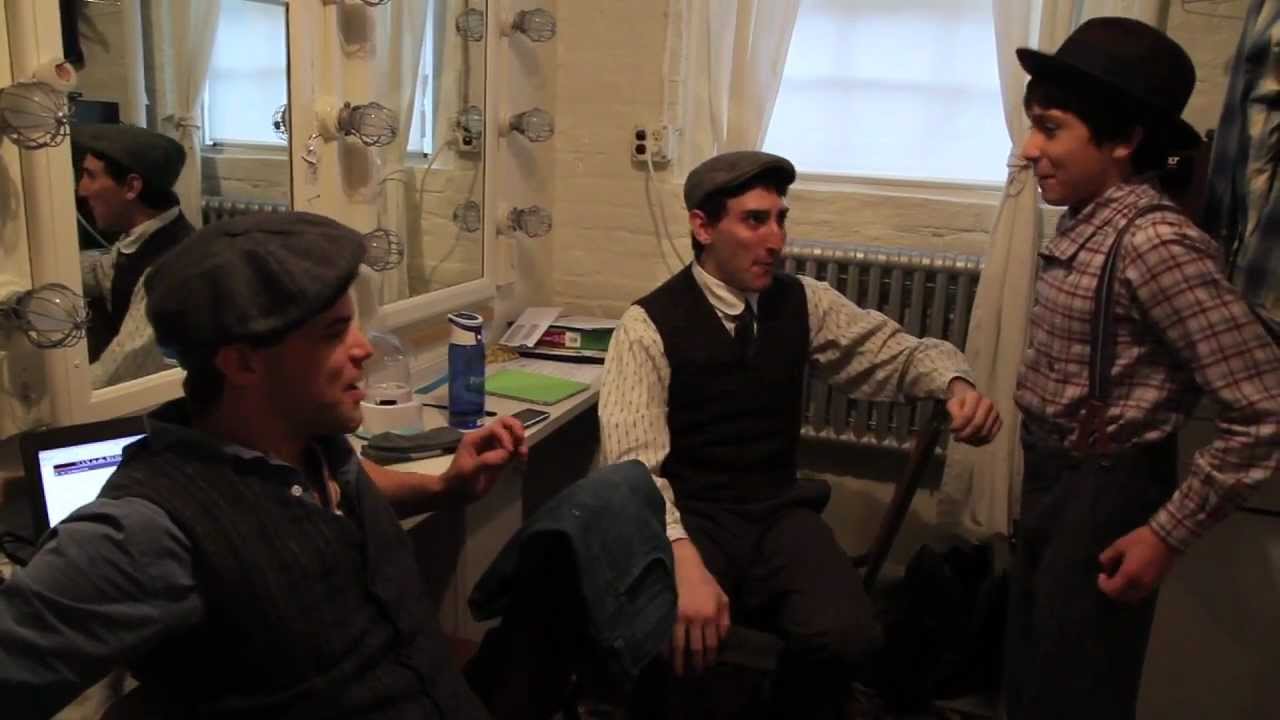In a cozy, cream-colored dressing room, bathed in the charm of the early 1900s, three males are captured in a lively conversation. Two men, donned in newsboy caps and period attire, sit comfortably, gazing with warm smiles at a young boy standing before them. The boy, around 13 or 14 years old, is dressed in a dapper top hat, suspenders, and a flannel shirt, evoking the nostalgic fashion of the 1920s or 1930s. Behind them, ornate mirrors adorned with unlit stage lights create a theatrical ambiance. The desk in front of the mirrors is cluttered with a mix of modern and personal items, including a laptop, iPhone, water bottles, and pens. A window with white curtains and a drawn shade lets in soft daylight, while a space heater stands against the wall, adding to the warmth of the scene. The room, likely backstage, hums with the anticipation of performance as the trio shares a moment filled with smiles and engagement.